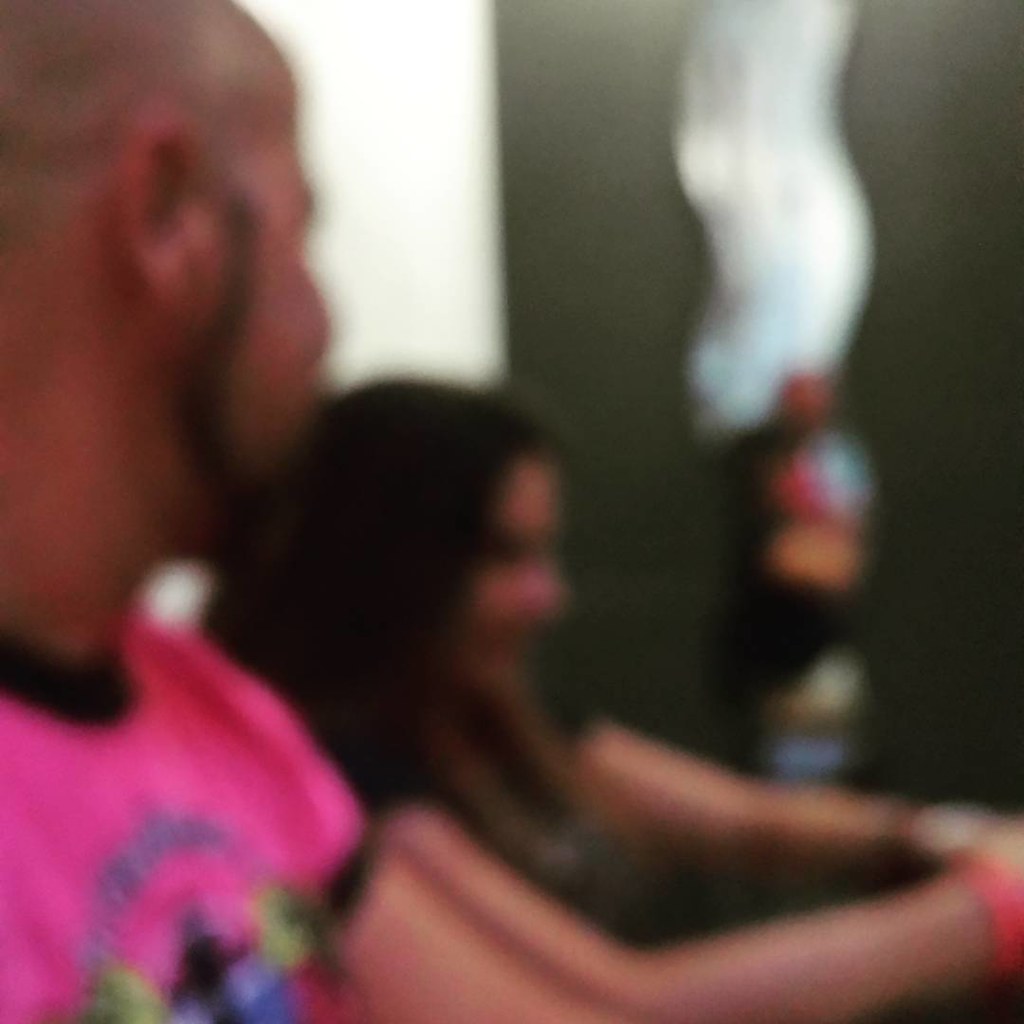This photograph, while out of focus, captures an intimate scene. In the foreground on the left, an African-American man with his head turned away from the camera is visible. He is wearing a pink t-shirt. The side of his face is partially seen, focusing particularly on his ear, as he looks away from the lens. Behind him, though still blurry, a woman with long dark hair can be seen sitting on the floor. Her knees are drawn up to her chest, and her arms are wrapped around them with her hands clasped together in front. The background remains even more indistinct, adding to the sense of depth and intimacy.